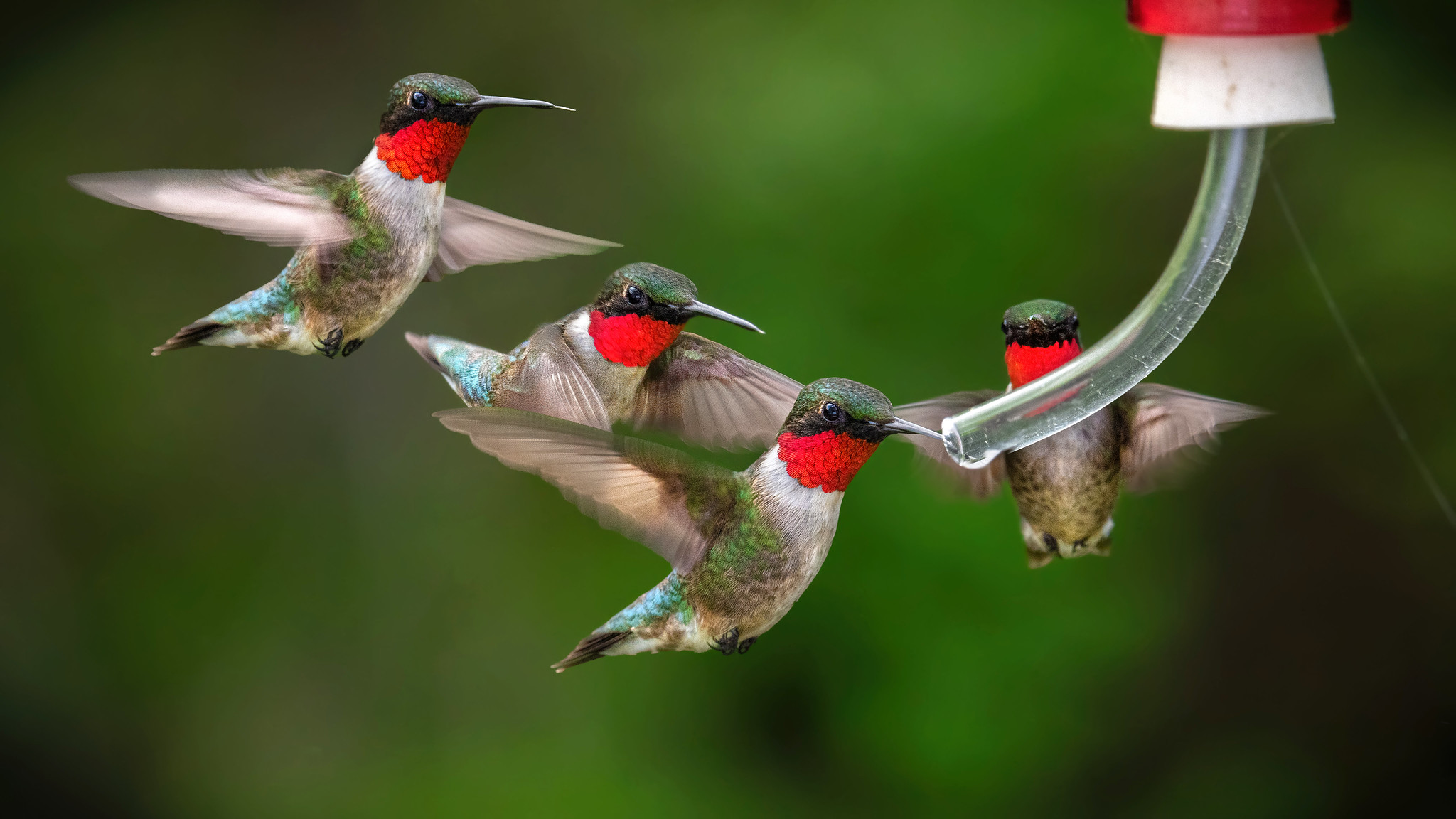This close-up outdoor photograph features four vibrant hummingbirds around a feeder, capturing a moment of frenetic energy as their wings blur with rapid movement. The birds share striking color patterns: green heads, black faces with long, black beaks, and red throats transitioning into white undersides. Their bodies display a mix of grayish-brown, iridescent greens, and subtle light blue tail feathers tipped in black, with spotted green and gray breasts. The feeder, detailed with a red top, white middle, and clear plastic tube curving downward, has one bird dipping its beak into the tube, while the other three hover nearby, seemingly waiting their turn. The out-of-focus green background suggests a lush, natural setting on a bright daytime.